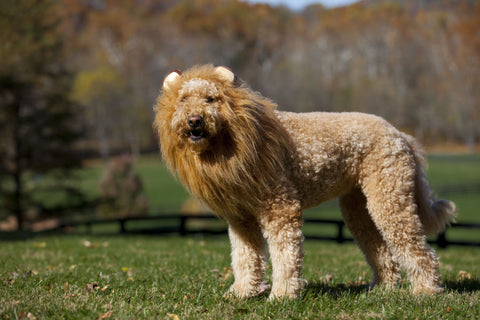In this very cute and humorous color photograph, we see an outdoor scene featuring a light tan and white dog, likely a labradoodle, adorned in a lion's mane costume. The scene is set on a grassy field full of green grass with scattered leaves, bathed in sunlight. The dog stands in the middle of the image, slightly angled to the right while looking directly into the camera at a three-quarter angle. He has a curly coat that is closely trimmed on his body, with a distinctive mane of long, flowing fur encircling his face, making him resemble a lion. His ears are tufted and perked forward, adding to the lion-like appearance. 

Behind the dog, the background features an unfocused view of mountains, a low black fence, and a tree to the left. There is also a stand of trees with golden vegetation and what seems to be a small wooden walking bridge, subtly blending into the scenery. The dog's black nose and calm, pleasant expression with its mouth slightly open give a warm and friendly vibe to the image, making it an engaging and charming representation of photographic realism.